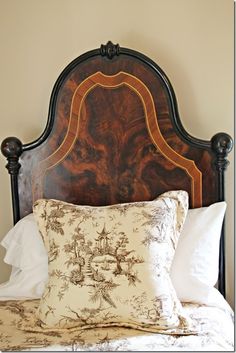The image is a color photograph taken indoors in portrait orientation, depicting a small, elegant bed set against a creamy magnolia-colored wall. Dominating the background is a Victorian-style headboard made of dark mahogany with inlaid lighter brown patterns and an arched, tubular frame. The headboard features intricate detailing at the center top, flanked by two spherical finials on either side.

In front of the headboard, there are multiple pillows: a square cushion with a cream cover, adorned with a bronze detailing and leaf pattern, and behind it, rectangular white pillows with plain pillowcases. The bed itself has beige linens with a matching vintage print that complements the Victorian aesthetic. The composition captures the sophisticated yet cozy setup, with the headboard casting a subtle shadow onto the wall, adding depth to the scene.